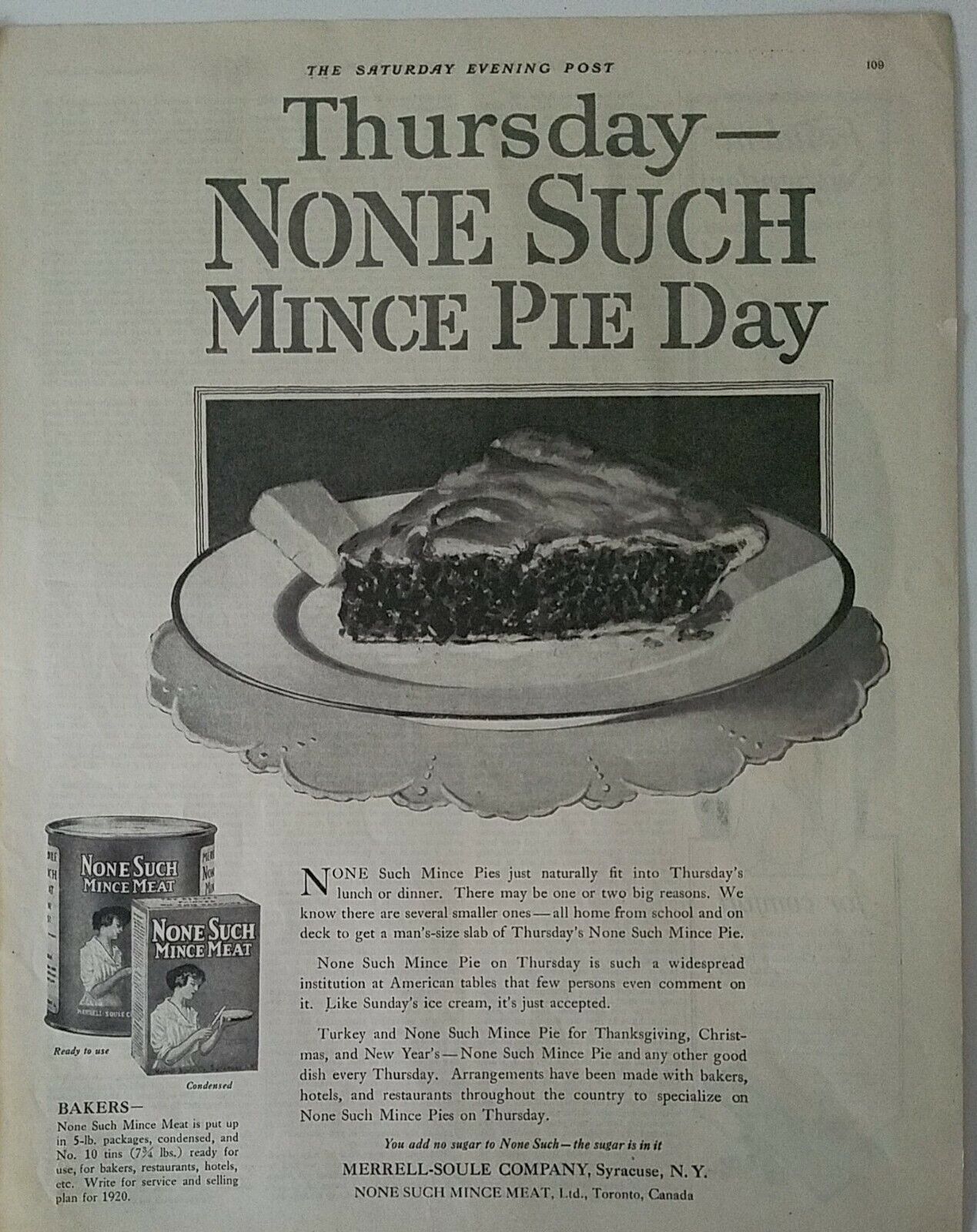This vintage black and white advertisement from the Saturday Evening Post features a detailed promotion for None Such Mince Pie. The ad is in good condition, with no visible tears, and appears to be a scan of a well-preserved newspaper or magazine page. At the top of the page, in small font, it reads "The Saturday Evening Post," followed by "Thursday" in larger font. Beneath that, in even larger letters, it says "None Such Mince Pie Day."

An illustration of a slice of mince pie, displayed on a white saucer resting on a doily, dominates the center of the ad. The pie wedge is detailed, with a pat of butter positioned on the left side of the plate. Below the image, three paragraphs describe the tradition and appeal of None Such Mince Pie, emphasizing its popularity at American tables especially on Thursdays, and outlining its convenience as the sugar is already included in the mince meat mix.

To the lower left of the page, there are images of the product packaging: a can of None Such Mince Meat featuring a woman holding a pie, and a box that likely contains the condensed version of the product. Small print at the bottom of the page provides manufacturing details, stating, "Merrill Soul Company, Syracuse, New York," and "None Such Mince Meat Limited, Toronto, Canada."

Overall, this advertisement highlights None Such Mince Pie as a staple for Thursday meals, likening its regular inclusion to other American traditions like ice cream on Sundays or turkey on Thanksgiving.